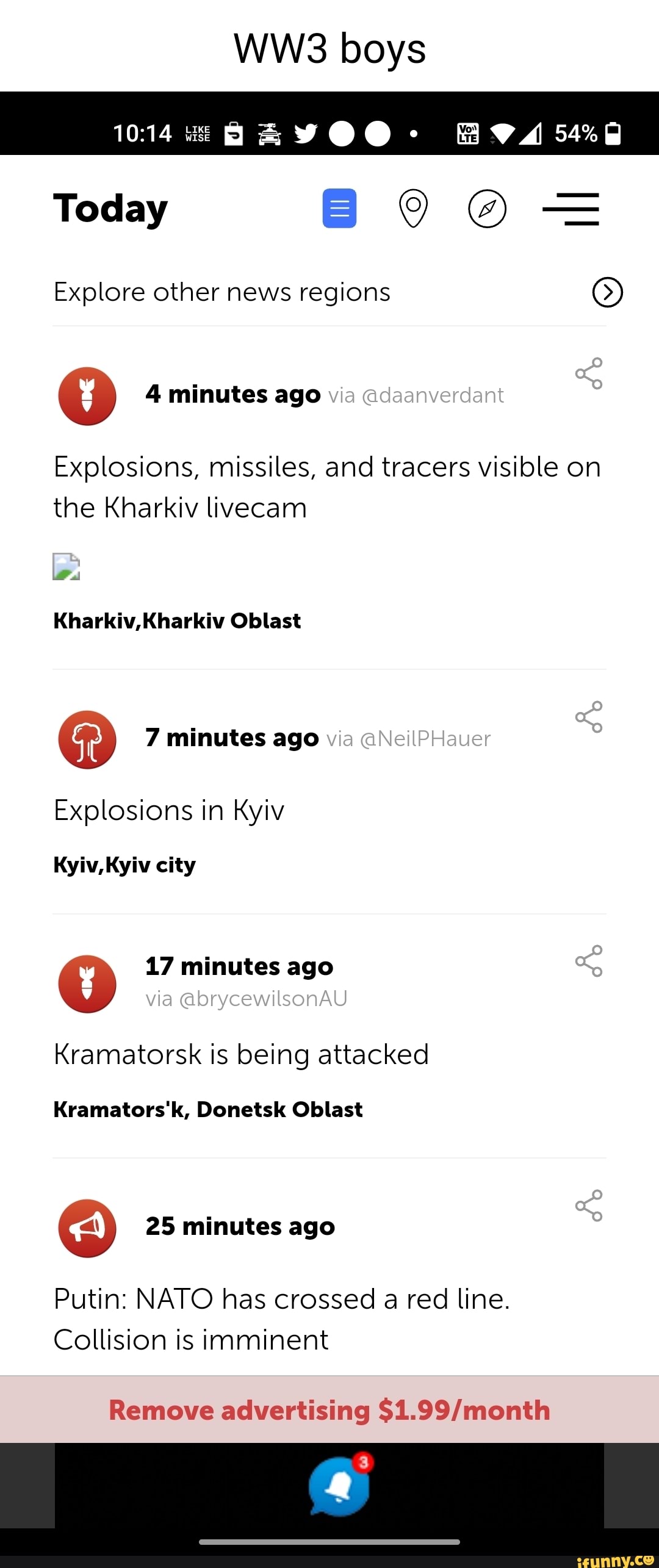The image appears to be a screenshot taken from a mobile phone, against a predominantly white backdrop. The top portion of the screen features a slim black bar with various icons and symbols. At the far left, a display reads "WW3 boys" while a thicker black bar beneath it spans the entire width.

In this black bar, white icons arranged from left to right include:
- A timestamp "10:14"
- A white box icon
- An icon resembling a white trash can
- Another indiscernible white icon
- A bird icon, likely representing Twitter
- A white circle
- Another white circle
- A white dot
- A gap
- Another white box
- Wi-Fi signal strength
- Phone signal strength
- A battery percentage "54%"
- A battery icon

Below this, the screen returns to a white backdrop with black text. On the left, the word "Today" is displayed, followed by a blue box containing three white horizontal lines. To the right is a black pen icon, a white circle with a black outline and compass hands inside, and three more black lines with the middle extending slightly to the left.

Further down, the text "explore other news regions" appears, flanked on the right by a white circle with a black outline and an arrow pointing right. Below this is a red circle with a white bomb icon pointing downwards, followed by "4 minutes ago via @daanverdan". Below this is the text "explosions, missiles, and tracers visible on the car key live cam".

A broken image icon appears next, with the text "car key, car key oh blast" below it. Continuing down, there's a red circle with a white mushroom cloud icon and "7 minutes ago via @neilphoward". Below that is "explosions in Keith" followed by "Keith, Keith city".

Further down, another red circle with a white bomb icon points downwards, followed by "17 minutes ago, via @BryceWilsonAU". The text "Chroma chromatorsk is being attacked" appears next, followed by "Chromatorsk, Donetsk Oblast".

Next is a red circle with a horn-like white icon, next to "25 minutes ago via @Putin: NATO has crossed a red line. Collision is imminent."

At the bottom, a light red, slightly pink bar spans the width of the screen with the text "remove advertising $1.99/month". In the center of this bar is a blue circle with a white bell icon, topped by a red circle with a white "3". Finally, in the lower right-hand corner in yellow text, it says "ifunny.com," suggesting this image is intended as a parody.